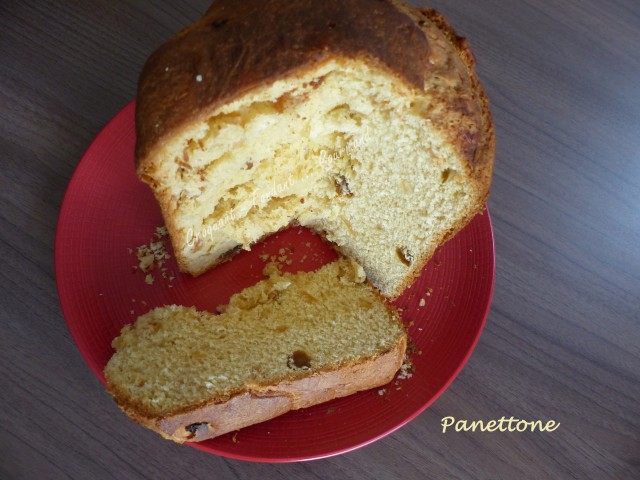The image features a large loaf of panettone, an Italian bread or cake, prominently displayed on a red, reflective plastic plate that rests on a textured, linoleum wood-style surface with brown diagonal lines. The panettone, which has a rich dark brown crust and a light yellow, cream-colored interior, is shown sliced with a piece cut off and laid flat in front of the main loaf. The sliced piece reveals the panettone's studded interior, showing bits of dried fruit, including what appears to be candied oranges and possibly nuts. The composition is complemented by some crumbs scattered on the plate. In the lower right-hand corner, the word "Panettone" is elegantly written in cursive with white lettering, adding a delicate finishing touch to the image.